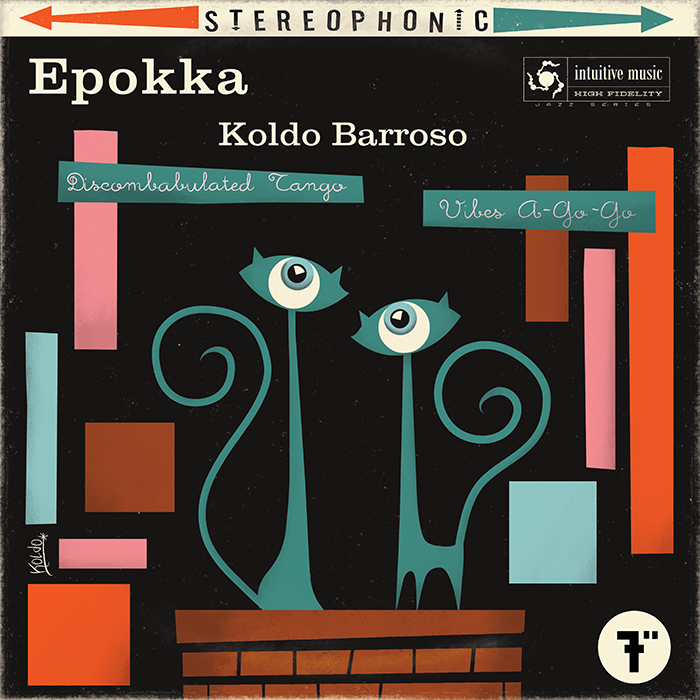This image is a detailed, stylized album cover with a black background that exudes a 60's art deco aesthetic. At the top, a white bar showcases the word "stereophonic" in black letters, flanked by an orange arrow pointing left and a teal arrow pointing right. Below, in large white text, the album prominently features the names "Epokka" and "Kolda Baraso." Additional text in a teal box reads "Discombobulated Tango" and "Vibes A-Go-Go," while a logo above declares "Intuitive Music, High Fidelity" alongside a small white emblem.

The main artwork consists of two whimsical, teal-colored cats with exaggeratedly long necks and tails that curl whimsically, topped with large single eyes. This playful imagery is complemented by various geometric patterns of rectangles and squares in hues of pink, orange, and blue scattered throughout the background. A white circle in the bottom right corner states "Seven Inch" in black letters, tying together this visually striking and musically indicative cover.